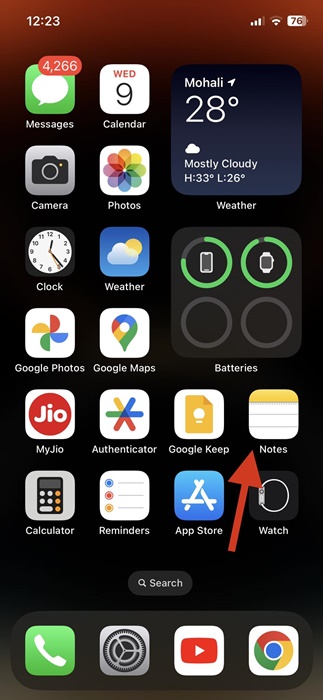A screenshot with a black background featuring a digital interface. The top section displays the current time as 12:23, alongside a battery indicator showing 76% charge. Below that, a blue square provides weather information, stating the location "Mahali" with a temperature of 28 degrees Celsius and mostly cloudy conditions, highlighted by a cloud icon. The high temperature for the day is noted as 33 degrees, with a low of 28 or 26 degrees. 

The screen is populated with various app icons, including Messages with a red notification circle displaying 4,266 messages, Calendar, Camera, Photos, Clock, Weather, Google Photos, Google Maps, My Geo, Authenticator, Google Keep, and Notes. A red arrow prominently points to the Notes app. Additional icons include Calculator, Reminders, App Store, Watch, and a gray oval search bar at the bottom featuring a magnifying glass icon. 

The screen's dock houses four icons: Phone, Settings, YouTube, and Google Chrome, neatly arranged for easy access.